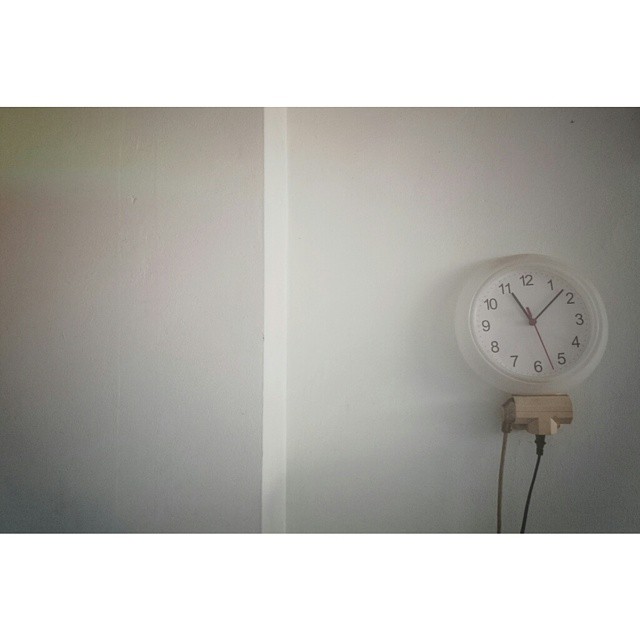The image displays a round, white-framed clock with a white face and black numbering from 1 to 12, positioned precisely at 11:07 AM/PM. The clock's hands, both hour and minute, are black, while the second hand is red and pointing towards the 27-second mark. This clock is mounted on a white, unfinished drywall wall, evidenced by visible white tape delineating the joint between two sections of drywall at the center. The photograph features top and bottom white borders typical of a 16:9 aspect ratio, likely indicating the image was captured using a wide-screen format camera. Below the clock, there is a small shelving unit, which also doubles as an electrical outlet hub. Two visible electrical plugs protrude from it, one brown (matching the base) and one black, providing a functional as well as a practical aspect to the scene.